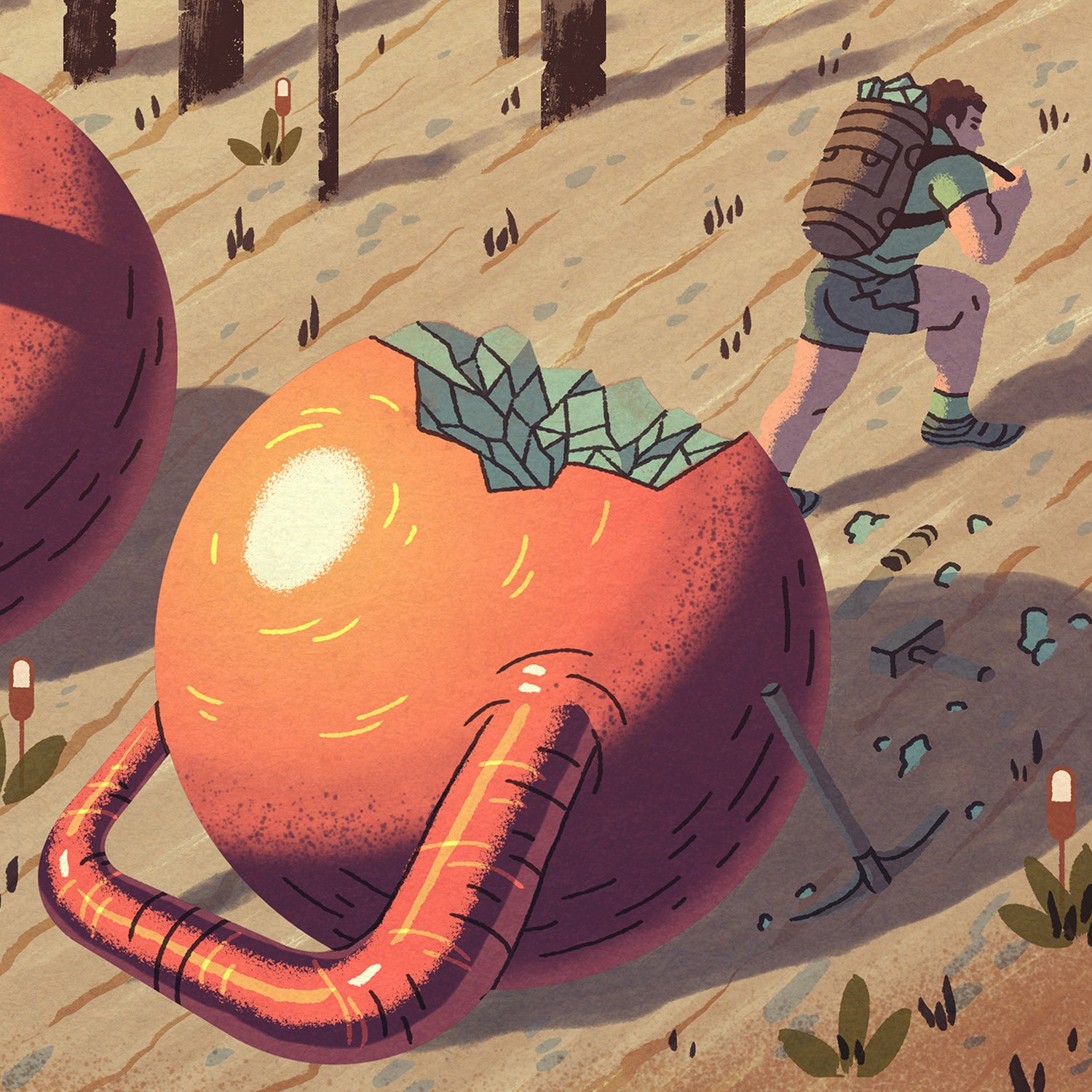The image is a vibrant, animated illustration depicting a Caucasian man hiking up a sandy hillside, characterized by a light brown color. He is wearing a light green shirt, dark green shorts, light green shoes, and carrying a large brown backpack brimming with green, diamond-like crystals. The hillside, sloping from the lower left to the upper right, features some plant life and is topped with tree trunks visible at the summit. The man appears to have mined these green crystals from a massive orange kettlebell positioned at the center of the scene, which has a handle near its base. Next to the kettlebell lies a pickaxe, indicating the kettlebell was broken open to extract the crystals inside. There's also a partial view of another red kettlebell in the upper left corner of the image, slightly clipped and illuminated by sunlight. The man, leaving the pickaxe behind, continues his trek up the hill with his backpack filled with the mined crystals.